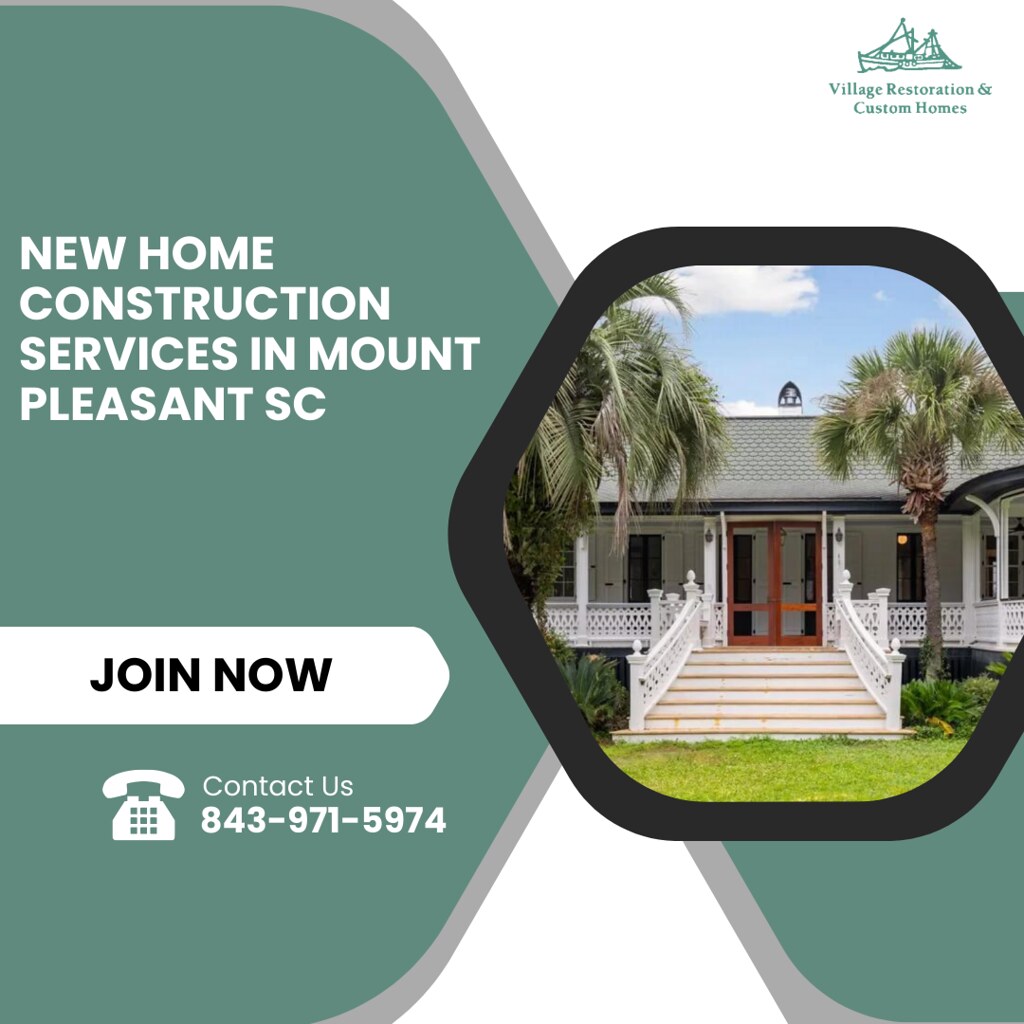This advertisement flyer for Village Restoration and Custom Homes, a home building company, features a vertical rectangular design with a distinct color scheme. The left side of the flyer has a green arrow shape, which is mirrored on the lower right, while the rest of the background is white. Prominently displayed in the center-right section is an image of a pristine white home with a green roof and a wide but shallow staircase leading to the front door. This home is framed by two palm trees and various bushes. The lush, green yard complements the house's plantation-like appearance, complete with a wraparound porch and shutters on the windows.

The top right corner of the flyer features the company's logo, which includes the text "Village Restoration and Custom Homes" along with a graphic of two sailboats. On the left side, the advertisement reads in bold white text: "New Home Construction Services in Mount Pleasant, SC." Below, it invites potential clients to "Join Now," providing a contact number: 843-971-5974. Various elements in circular designs, including a phone icon, emphasize the company's commitment to customer service and new home construction services in the specified region.